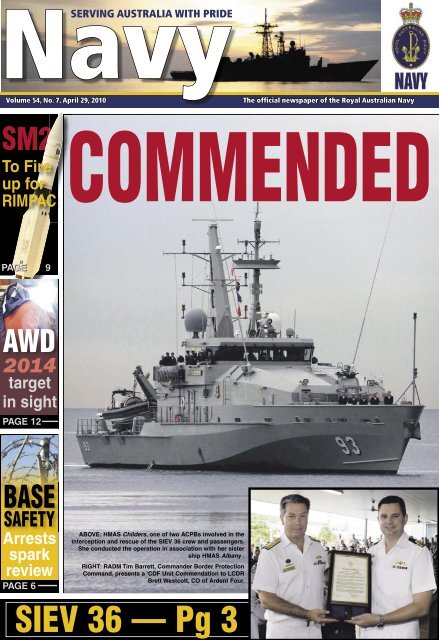This image depicts the cover of the **official newspaper of the Royal Australian Navy**, titled "Navy," specifically Volume 54, Number 7, dated April 29, 2010. Dominating the cover is a striking **black-and-white photograph of a large Naval ship**, prominently featuring the number 93. The ship is equipped with a substantial upper deck and numerous antennae spearing upwards. 

At the top, the headline reads, "Serving Australia with Pride," followed by "Navy" rendered in substantial white font against a blue backdrop, accompanied by a sunset image of another Navy ship. Just to the right of this title is the Navy's emblem, affirming the magazine's authoritative source.

In bold red font, the word "Commended" spans across the center of the cover, drawing immediate attention to the commendation theme. 

On the lower right corner, there is a **photo of two Caucasian men in white Navy uniforms** beaming while holding a plaque. Various headlines are dispersed on the left side enclosed in rectangles, including:
  - "SM2 to fire up for RIMPAC"
  - "AWD 2014 Target In Sight - Page 12"
  - "Base Safety Arrest Sparks Review - Page 6"
  - "SIEV 36 - Page 3"

Additional minor black text is present below the main ship image but is too small to be read clearly. The magazine's diverse color palette includes black, white, grey, brown, yellow, blue, and red, adding vibrance to the professional and patriotic presentation.